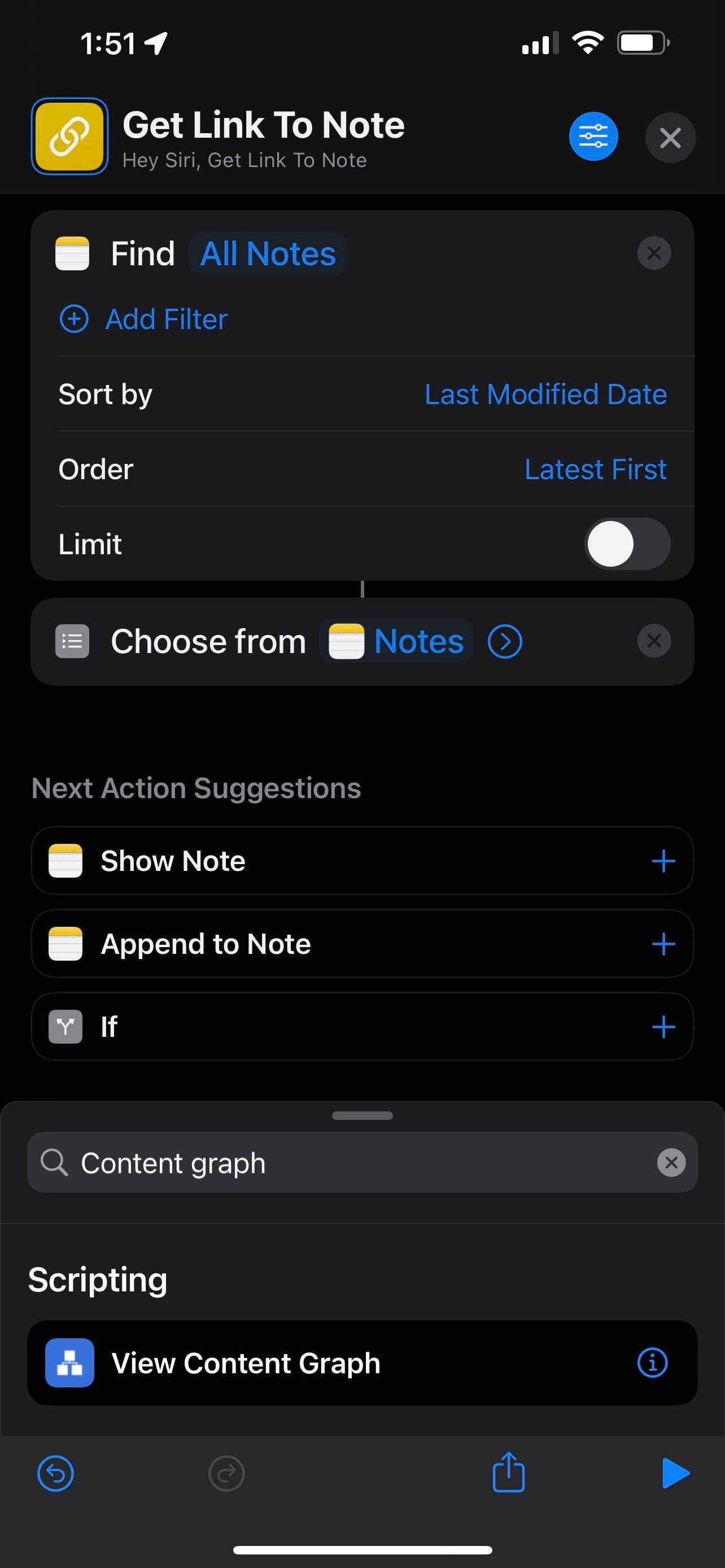The image is a detailed screenshot of the Shortcuts app on an iPhone. At the top left corner, the time reads 1:51, while the right corner includes the data, WiFi, and battery icons. The shortcut featured in the image is titled "Get Link to Note." Below the title, the phrase "Hey Siri, get link to note" indicates the voice command required to activate the shortcut. The shortcut workflow consists of finding all notes sorted by the last modified date in descending order, with no limit set. The phrase "Choose from Notes" suggests an action within the workflow. Next action suggestions include "Show Note," "Append to Note," and a conditional "If" statement. At the bottom of the screen, a search box contains the text "Content Graph." To the left of the search box, the option "Scripting" is visible. Under the search box is a button labeled "View Content Graph."